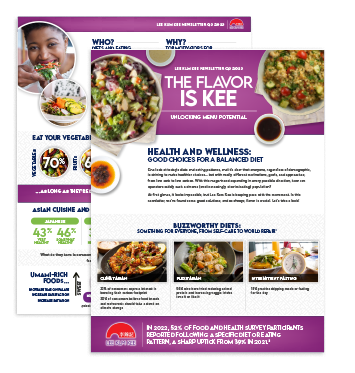The image features two overlaid advertisements or web pages, creating a visually complex scene. 

The first ad displays a vibrant purple header adorned with various food images. On the left, there's a white bowl containing a colorful salad with green, red, yellow, and orange elements. To the top right of the header, a dish of yellow grains mixed with red tomatoes and green vegetables is visible. Overlaying this header, white text reads, "The flavor is key. Unlocking menu potential," with additional blurred white text above it that's unreadable. Scattered around the header are three small white sauce dishes: a pale yellow sauce positioned just up and to the right of the salad, a brown soy-sauce-like condiment down and to the left of the grain dish, and an orange dish with a brown center located just below the salad.

Beneath the purple header, a section with a white background features blue text that announces, "Health and wellness. Good choices for a balanced diet." Two paragraphs of black text are situated below this line, but they are too blurry to be decipherable.

The bottom section of the image showcases another layer of information set against a 45-degree-angled gray square pattern. Dark blue text at the top states, "Buzzworthy diets. Something for everyone. From low-carb to world," although the complete message is partially obscured due to blurring. Beneath this, three small images are presented: on the left, a shrimp dish in a black bowl; in the middle, another shrimp dish with additional green, red, and orange components, also in a black bowl; and on the right, a yellow and white alarm clock alongside a white dish filled with green and orange food.